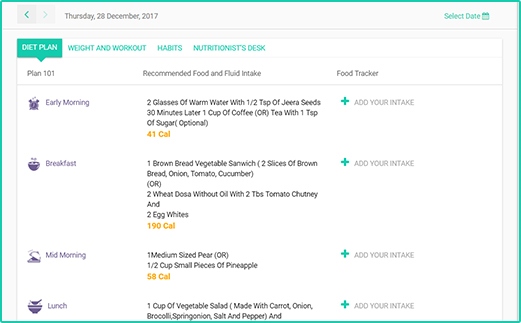The image depicts a detailed diet plan interface dated December 28, 2017. At the top, there is a date display, with an arrow that allows users to navigate back to previous dates, and a date selection button on the right side for accessing the calendar. The interface is divided into various sections, with a green button labeled "Diet Plan" at the center. To the right of this button, there are three additional buttons for different functions: "Weight and Workout," "Habits," and "Nutritionist Desk," the latter likely providing a feature to ask questions about healthy food choices and recipes.

Below the "Diet Plan" heading, there is a labeled column titled "Plan 101," which details the daily eating schedule, broken down into segments such as early morning, breakfast, mid-morning, and lunch. To the left of each segment, there is a corresponding icon. The middle column outlines the recommended food intake for each time slot. For instance, in the early morning section, the plan advises consuming two glasses of warm water mixed with half a teaspoon of Jara seeds, followed 30 minutes later by one cup of coffee or tea with an optional teaspoon of sugar. It also suggests an orange, which amounts to 41 calories.

The right-most column features a food tracker with a green plus sign, which enables users to add their food intake. The breakfast section recommends a brown bread vegetable sandwich, consisting of two slices of brown bread filled with onion, tomato, and cucumber. For the mid-morning snack, it suggests a medium-sized pear or half a cup of pineapple. For lunch, the plan includes one cup of vegetable salad with assorted chopped vegetables.

This comprehensive interface offers a structured and interactive way to manage daily dietary habits with personalized suggestions and tracking capabilities.